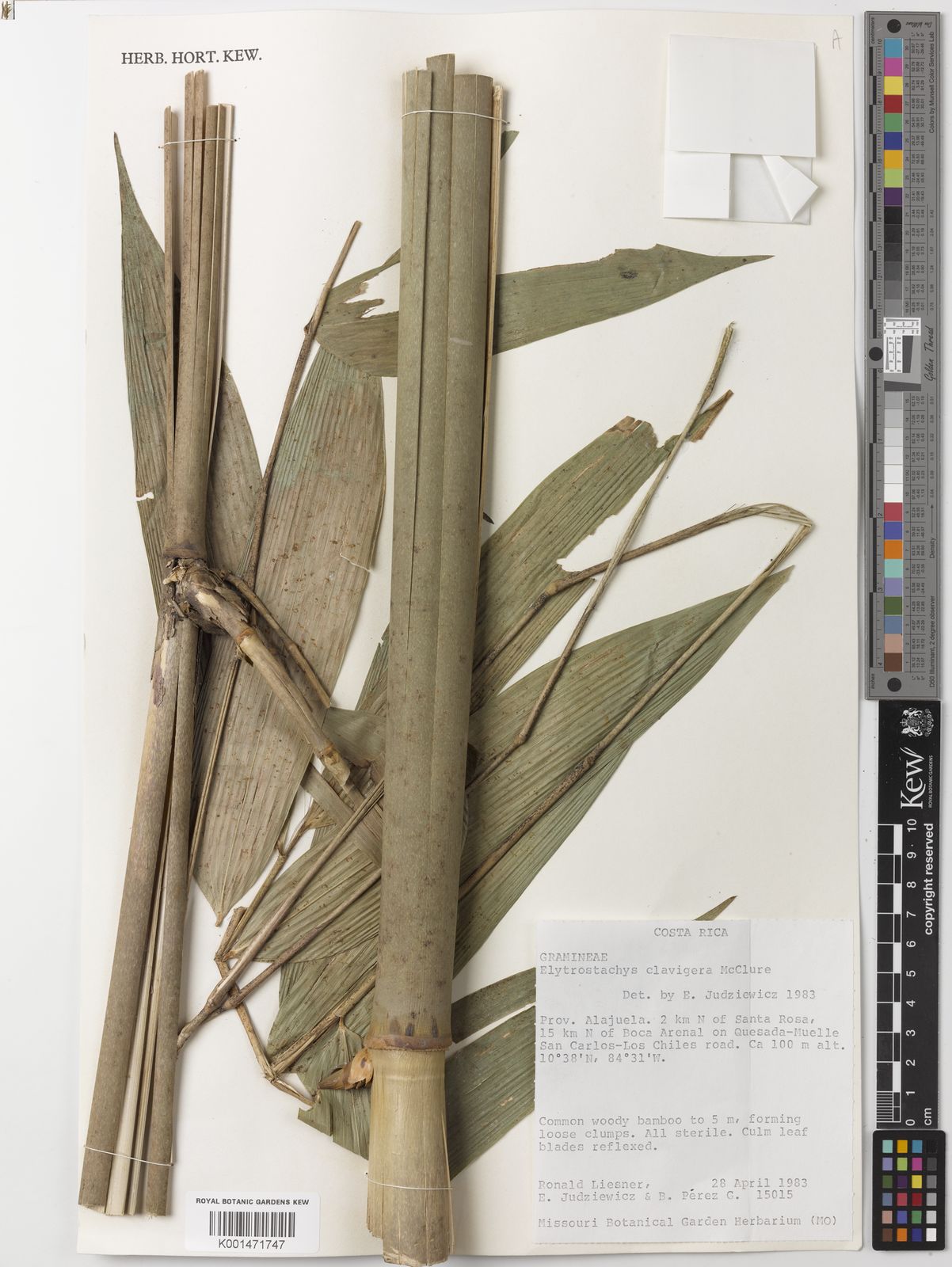The image depicts an off-white sheet of paper, prominently displaying a specimen of plant life that appears brownish in color, attached to the left side. Above this plant specimen, the label "Herb Hort Q" is clearly visible. A ruler is positioned along the right side of the paper, measuring it, and just in front of the ruler is a folded patch of paper. Between the ruler and the plant specimen, there is a smaller piece of paper inscribed with "Costa Rica" and additional text beneath it. The bottom-left corner of the paper contains a barcode. On the top right, there is another piece of folded paper. On the far right edge, there is a color bar displaying a range of colors from blue, purple, yellow, dark red, green, blue, orange, and different shades of gray, akin to a selection tool used in digital design or graphic art software. The overall setting gives the impression of a botanical or scientific documentation, potentially for research or educational purposes.